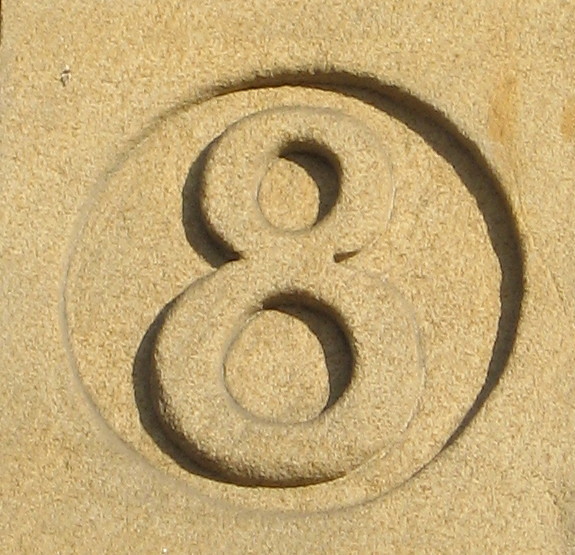This square-format, color photograph showcases an aerial view of a tan-colored stone field featuring an intricately carved number 8, reminiscent of a crop circle. The photograph captures a zoomed-in perspective, making the engraved 8 the focal point. The number 8 is carved inside a larger circular depression at the center of the image, with both the circle and the number casting subtle shadows, suggesting light coming from the right. The stone field exhibits a textured surface, with dark yellow streaks accentuating the top-right portion of the image, adding depth and dimension. The shading within the carved details further enhances the three-dimensional appearance of the number 8 and its surrounding circle.